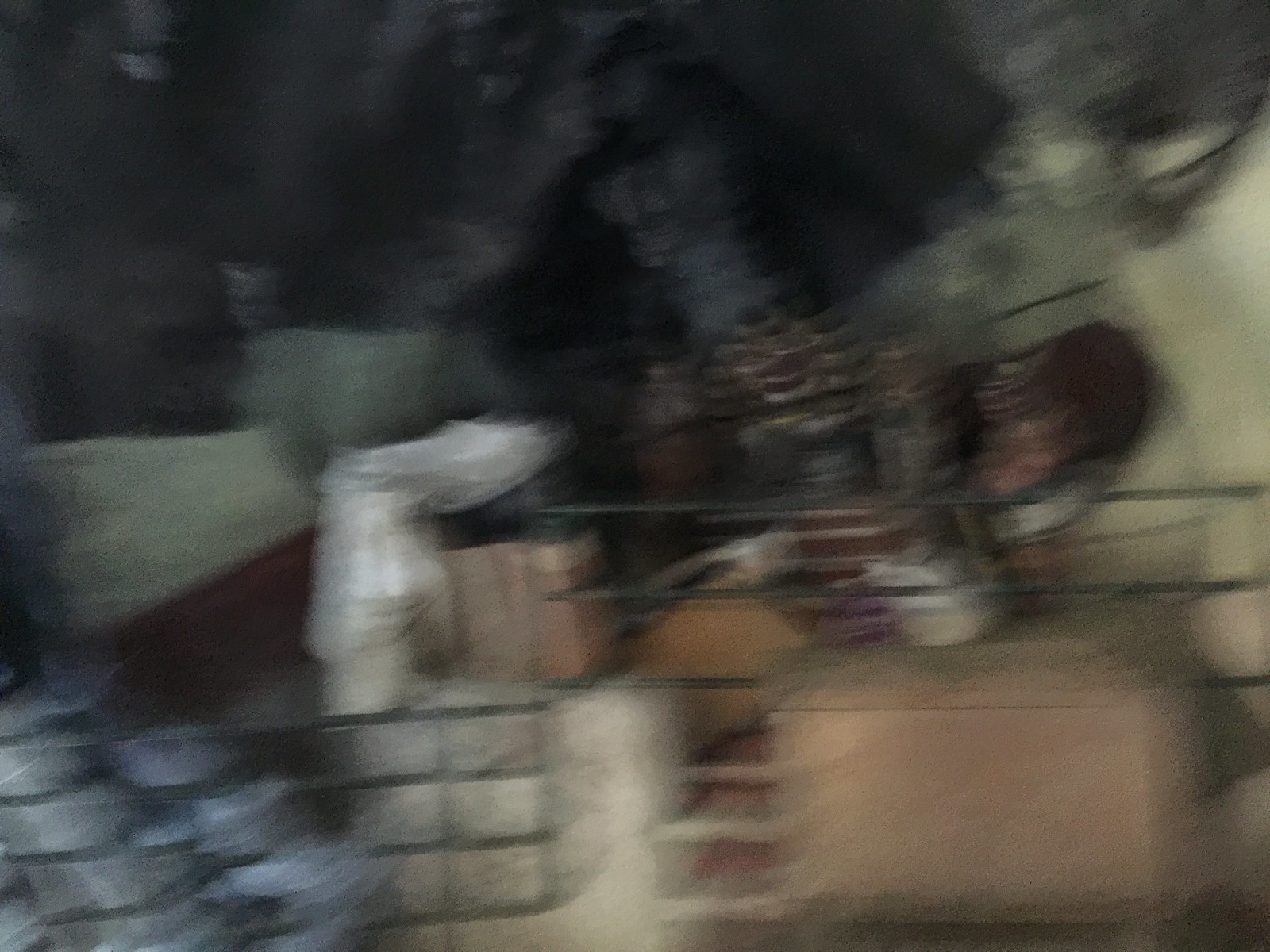The image is exceptionally blurry, making it challenging to discern whether the setting is indoors or outdoors. The color palette is predominantly composed of dark, muted tones, which blend together in a way that obfuscates the scene. The upper portion of the image features a mix of black and gray hues, punctuated by long black streaks adjacent to what appears to be a gray head or neck area. To the right side of the image, there is a cluster of tan objects blurred together. 

In the center or perhaps slightly to the left, a few cream-colored throw pillows can be faintly distinguished. There also seems to be a collection of boxes in the middle of the image, interspersed with gray, wiry crates that have a see-through appearance due to the bars running across them. Additionally, a white plastic or white-colored box is situated beneath the crates. The overall blurriness of the picture makes it nearly impossible to pinpoint the exact elements or the context of the scene.